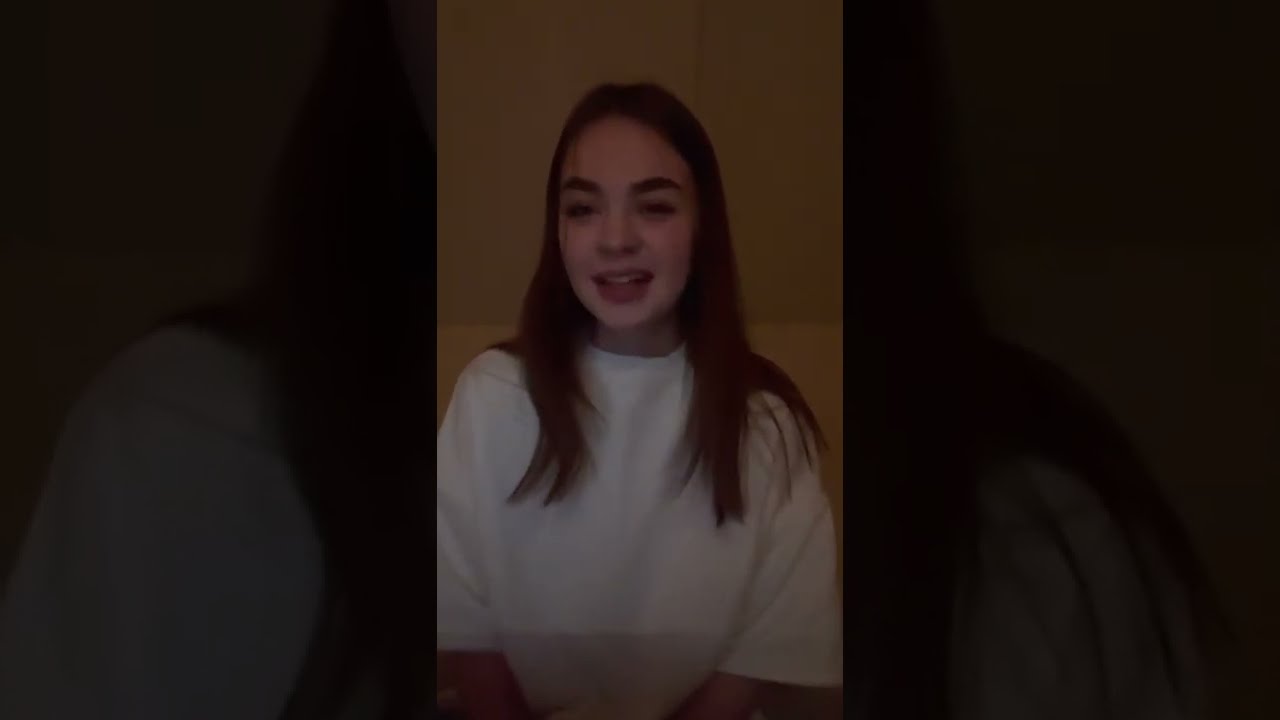In the center of the horizontally aligned rectangular picture is a young woman with long, straight, dark brown hair, pulled over her shoulders and parted in the middle. She is smiling warmly, revealing her teeth, which are accentuated by what appears to be red lipstick. Her thick brown eyebrows stand out against her smooth complexion. She is wearing a slightly oversized, short-sleeve, white t-shirt with wide cuffs around her elbows. Her hair falls past her shoulders, with a few strands of hair draping down over her right eye. The woman appears to be seated, with her arms possibly folded on her lap, though her hands are not visible below the elbows. The backdrop is a plain tan wall, suggesting an indoor setting with dim, yellowish lighting, possibly from a nearby lamp.

Flanking the central image are two narrower, vertical close-ups of her. On the left, a closeup captures a darker, blurrier version of her right shoulder and hair. On the right, another darker, blurrier closeup shows the left side of her shoulder and hair. The overall effect gives a sense of depth and focuses attention on her serene and content expression despite the dim lighting.